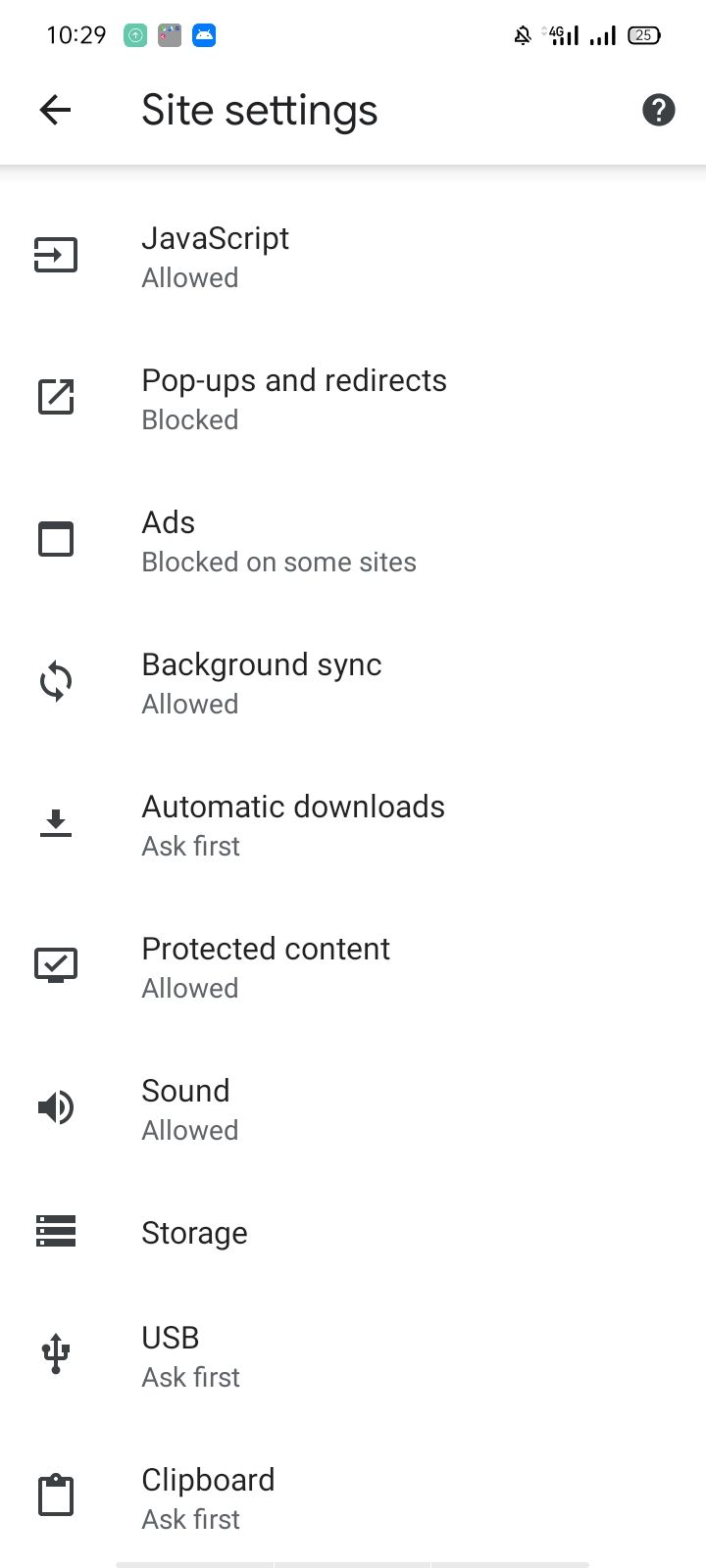This screenshot captures the display of a settings menu on a mobile phone, outlined against a white background with black text. In the upper left-hand corner, the time reads "10:29" alongside three boxes: a green one, a grey one, and a blue one with white writing that is too small to discern. The upper right-hand corner shows two signal strength indicators for different SIM cards, along with a battery icon and a bell icon.

Central to the screenshot is the title "Site Settings" in black, flanked by a back arrow on the left and a question mark enclosed in a black circle on the right. Below this is a thin horizontal line that spans the width.

The settings list displays various options, each with small black and white icons to their left. The list includes:
- **JavaScript:** Allowed
- **Pop-ups and redirects:** Blocked
- **Ads:** Blocked on some sites
- **Background sync:** Allowed
- **Automatic downloads:** Ask first
- **Protected content:** Allowed
- **Sound:** Allowed
- **Storage:** Nothing listed
- **USB:** Ask first
- **Clipboard:** Ask first

Each listed setting has a corresponding icon: 
- **JavaScript** (not described in the text), 
- **Pop-ups and redirects** (not described),
- **Ads** (not described),
- **Background sync:** A simple reload icon
- **Automatic downloads:** A down arrow with a horizontal line
- **Sound:** A standard sound icon
- **Storage:** Three bars
- **USB:** Resembling a three-pronged fork
- **Clipboard:** A clipboard image

Underneath the list is another grey horizontal line, extending about halfway across the screen. The icons for the settings are simplified, primarily black and white, with most, like the Background sync icon and the USB icon, being square-shaped.